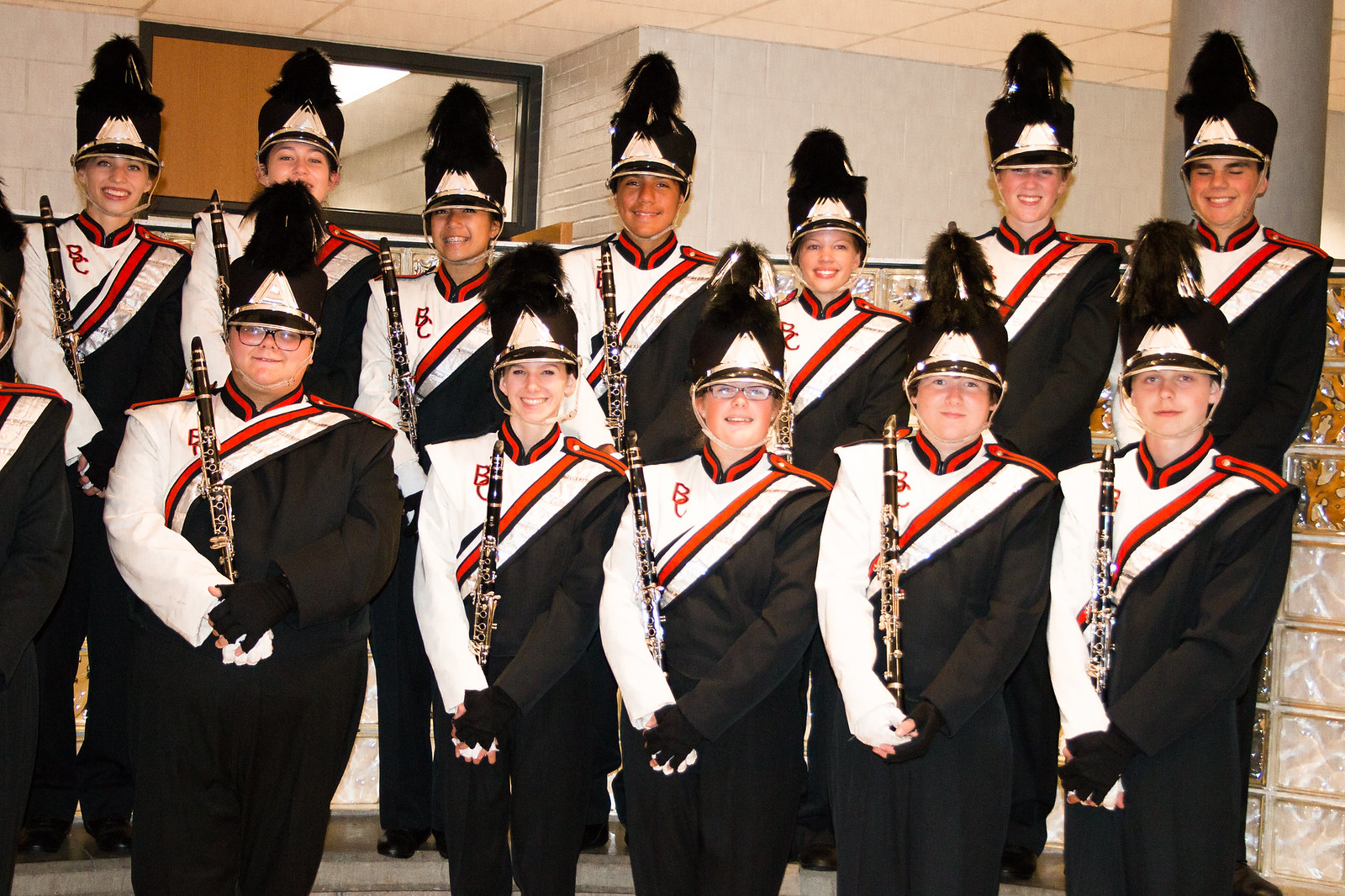This photograph captures a high school marching band posed in an indoor school setting. The room features distinctive white tile roofing and a light grayish-white brick wall, accented by a substantial silver pillar. The space also includes a transom window above a door, half transparent and half solid with dark yellowish brick framing. 

The band is arranged in two rows: the back row consists of seven members standing on a riser, while the front row comprises six members. Each musician is dressed in a striking uniform that blends black, white, and red. The uniforms feature a predominantly black base with a white left shoulder and sleeve, contrasted by red striping and BC embroidery on the left shoulder. The ensemble is completed with elaborate black and white hats adorned with large black feather plumes.

All band members are holding their instruments, which appear to be wind instruments such as flutes or clarinets, in a uniform manner - vertically along their right shoulders, with both hands resting near their stomach region. Additionally, their gloves feature an alternating color scheme of black on one hand and white on the other. The group, composed of both boys and girls, uniformly smiles and gazes directly at the camera, exuding happiness and camaraderie.